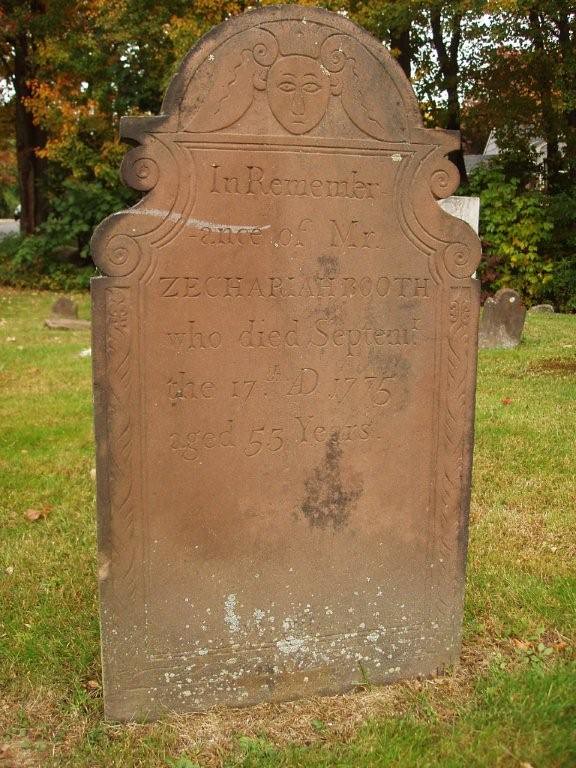**Caption:**

A vertical photograph capturing an aged gravestone standing in the center of an old cemetery. The weathered headstone, a mix of tan, beige, and gray hues, is inscribed with the words "In remembrance of Mr. Zeke Hi Booth, who died September 17th, age 55 years." The gravestone, which stands upright, dominates the image, framed by green grass at the bottom and towering trees in varying shades of green and brown at the top. The setting is an outdoor cemetery, with the solemn atmosphere enhanced by the subdued and earthy color palette, and the photograph's vintage appearance adds a timeless feel to the scene.